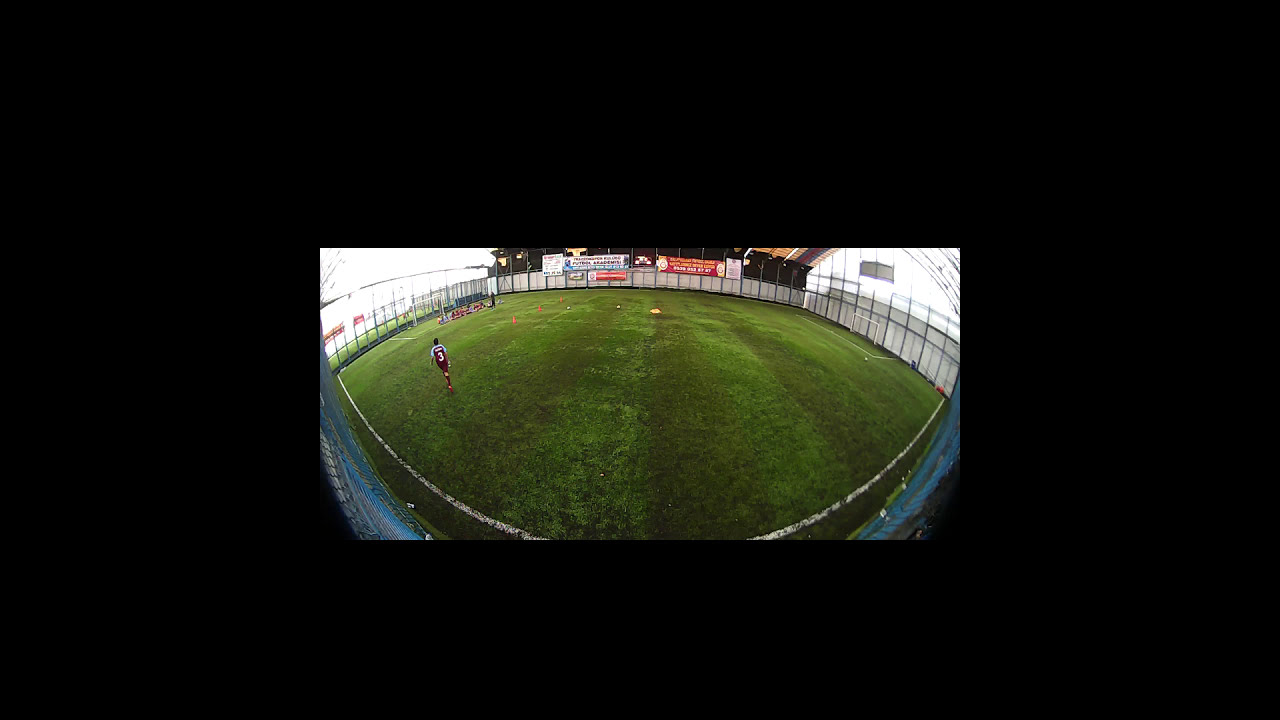The image captures an almost empty soccer field from the perspective of a spectator high up in the bleachers. Taken with a fisheye lens, the scene is notably distorted, giving a circular appearance where the center looks closer, and the edges appear farther away. The lush grass field features alternating horizontal stripes of lighter and darker green. Encircling the field is a chain-link fence adorned with unreadable advertisement signs.

In the distance on the left side, a few individuals in soccer uniforms are seated near the goalpost. Prominently, a single player wearing a purple jersey with a white number three and black socks with orange stripes is walking away from the camera toward the center-left of the field. Near the goal, several soccer balls are lined up, indicating he might be preparing for shooting practice. Additionally, there are pylons placed before the goal line, adding to the structured practice setup.

Overall, the serene atmosphere and composition draw focus to the lone player's quiet preparation against the vast, encircling fence and distant signs, accentuated by the uniquely distorted fisheye perspective.